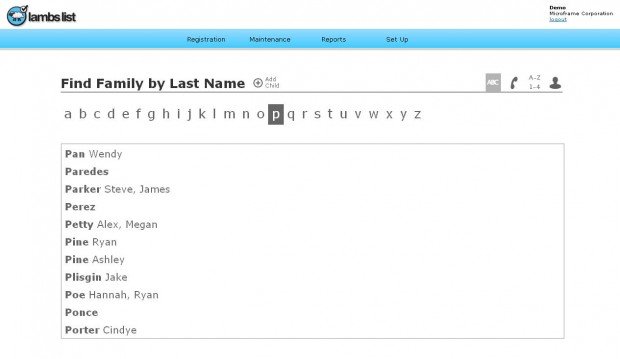The image is a screenshot of a website interface labeled "Lambs List" at the top. The title "Lambs List" appears in black text, accompanied by a blue circle housing a white sheep icon with a black checkmark. Below this header, there is a blue navigation bar featuring black sub-menus labeled "Registration," "Maintenance," "Reports," and "Setup."

At the top, some smaller black text items are visible but are too small to be legible. Directly beneath the blue bar, there is a search field labeled "Find Family by Last Name," next to an "Add Child" button with a gray circle. To the right, there are various gray icons including "ABC," a phone icon, "A to Z," "1 to 4," and a floating head and shoulders icon.

Further down, the letters A through Z appear in gray, indexing a white box filled with listed names. These names, displayed in black or gray text, include:

- Pan Wendy
- Herades
- Parker Steve James
- Perez
- Petty Alex Megan
- Pine Ryan
- Pine Ashley
- Plagueskin Jake
- Poe Hannah Ryan
- Ponce
- Porter Cindy

The list is separated by thin gray lines, and although the top of the image appears somewhat pixelated, the overall image quality is decent.